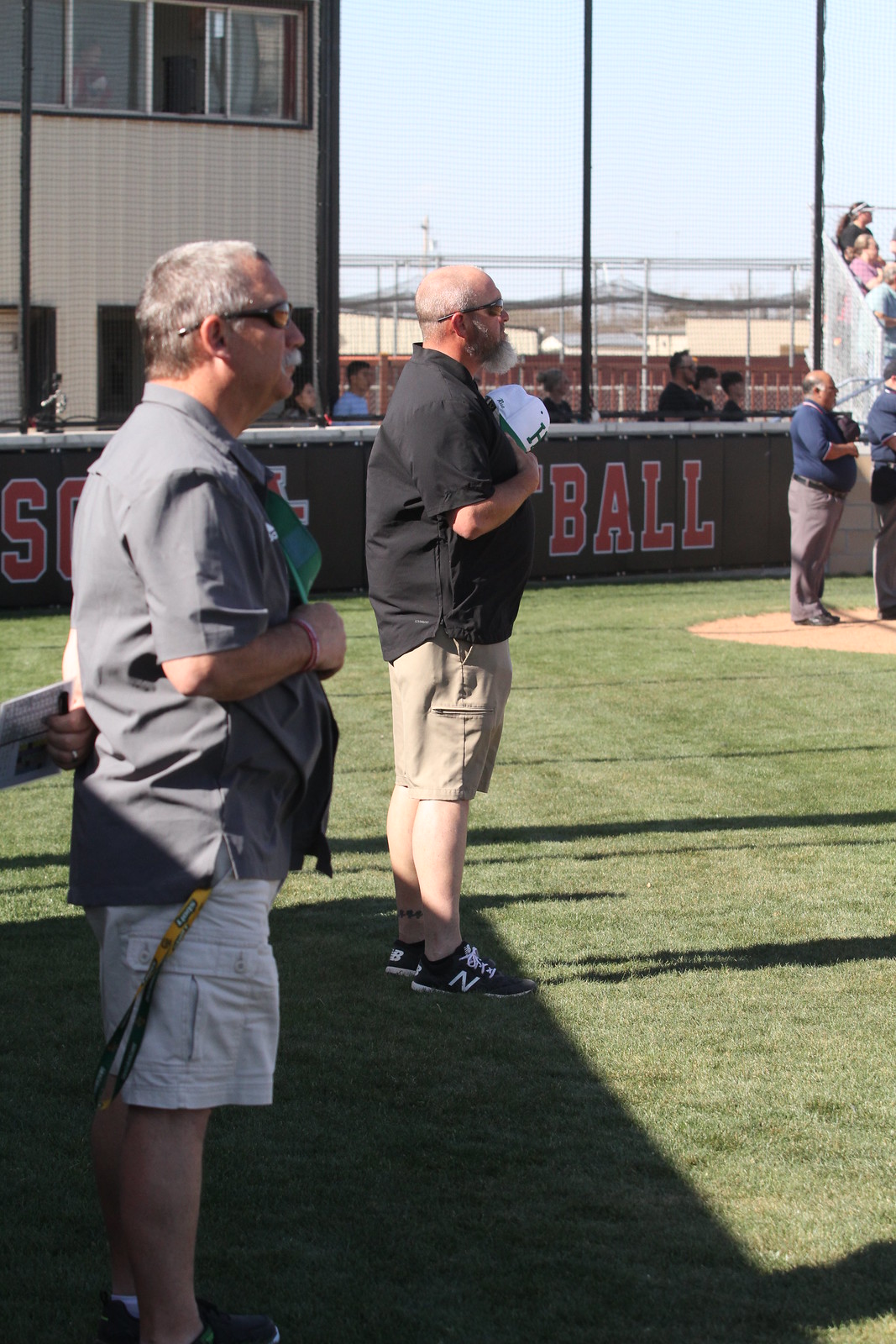The photograph captures a serene moment at a baseball field, likely during the prelude to a game, as individuals stand in reverence for the National Anthem. The image shows a group of people positioned on the lush grass, adjacent to a small dirt area, possibly near the pitcher's mound or the end of the infield. Framing the field is a padded outfield wall, beyond which stands a mix of spectators, also facing forward with their hands over their hearts.

Prominently featured are two men, entirely visible, both dressed in polo shirts—one dark and one black—with khaki shorts, each holding their hats to their chests in a gesture of respect. Further into the background, protective netting rises above the wall, ensuring the safety of those beyond. Behind this netting, there’s a building that likely houses restrooms or facilities for the announcers and scorekeepers.

In the top right-hand corner, the image reveals the edge of the stands filled with spectators, all poised in anticipation of the game. The skyline is dotted with additional structures and crisscrossed by power lines, perhaps hinting at the presence of batting cages. This detailed scene collectively evokes the anticipation and solemnity of the moment before a community engages in the timeless ritual of America's pastime.